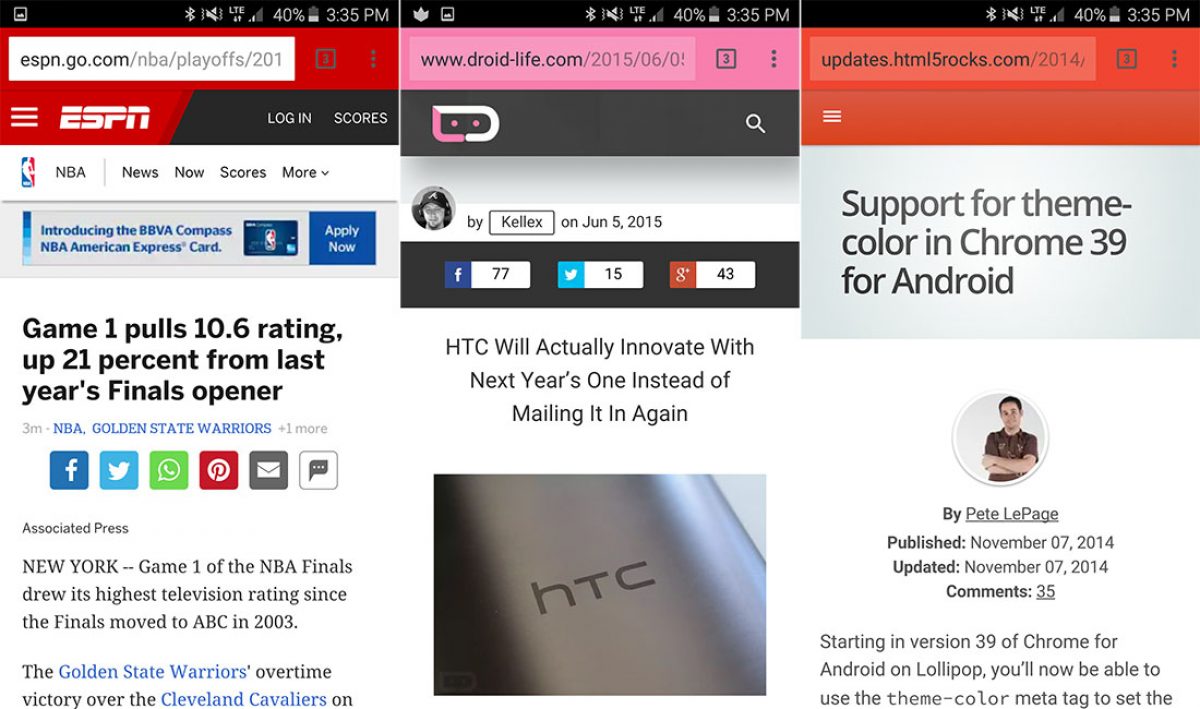The image consists of three successive screenshots taken from the same phone, all captured at 3:35 PM with a battery level of 40%. Each screenshot features the top bar showing time and battery status, with each representing a webpage from a different source. The three sources displayed are espn.com, droid-life.com, and updates.html5rocks.com, presented from left to right.

1. **ESPN Website (Leftmost Screenshot)**:
    - The screenshot is from ESPN and features a distinctive red border with white text.
    - The article headline reads: "Game 1 pulls 10.6 rating, up 21% from last year's finals opener" in bold black text.
    - The article begins with "New York" and states, "Game 1 of the NBA Finals to its highest television rating since the finals moved to ABC in 2003," followed by additional text not fully visible in the screenshot.

2. **Droid Life Website (Middle Screenshot)**:
    - The screenshot displays an article by Kellix, posted on June 5th, 2015.
    - The headline reads: "HTC will actually innovate with next year's one instead of mailing it in again."
    - An image of an HTC device appears below the headline, showing a silver cylinder design.

3. **HTML5 Rocks Website (Rightmost Screenshot)**:
    - This screenshot features an article about Chrome development for Android.
    - The headline reads: "Support for theme color in Chrome 39 for Android," authored by Pete LePage and published on November 7th, 2014.
    - The article begins with: "Starting in version 39 of Chrome for Android or on Lollipop, you'll now be able to use the theme color and Meta tag to set..." before the text gets cut off.

Each screenshot captures a specific moment across different websites, reflecting the diversity of content accessible through mobile devices.